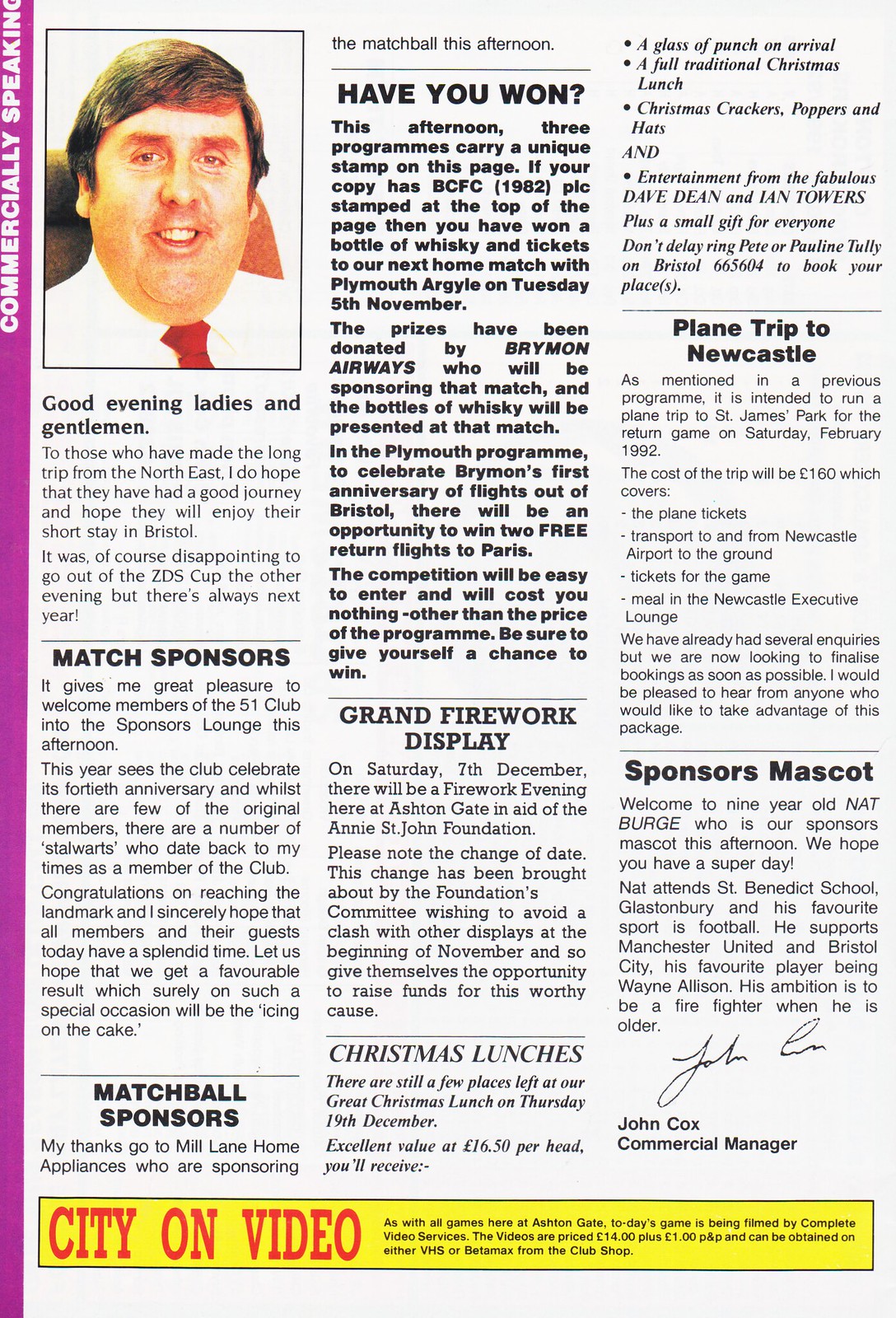This detailed image resembles a page from a newspaper or bulletin. In the top-left corner, there's a photograph of a man with short brown hair. He is wearing a white button-down shirt and a red tie, and the picture shows his head, neck, and part of his shoulders. The page is filled with various columns of text in different fonts and styles, all set against a white background with black text. The headlines of some articles include "Match Sponsors," "Match Ball Sponsors," "Have You Won?", "Grand Firework Display," "Plane Trip to Newcastle," "Sponsors Mascot," and "Christmas Lunches." On the left-hand side of the page, there is a purple vertical strip that reads "Commercially Speaking." At the bottom of the page, there's a yellow horizontal strip with red text that says "City on Video." The article content appears to be related to sports events, promotional announcements, and festive activities, all presented in a newspaper-style format.